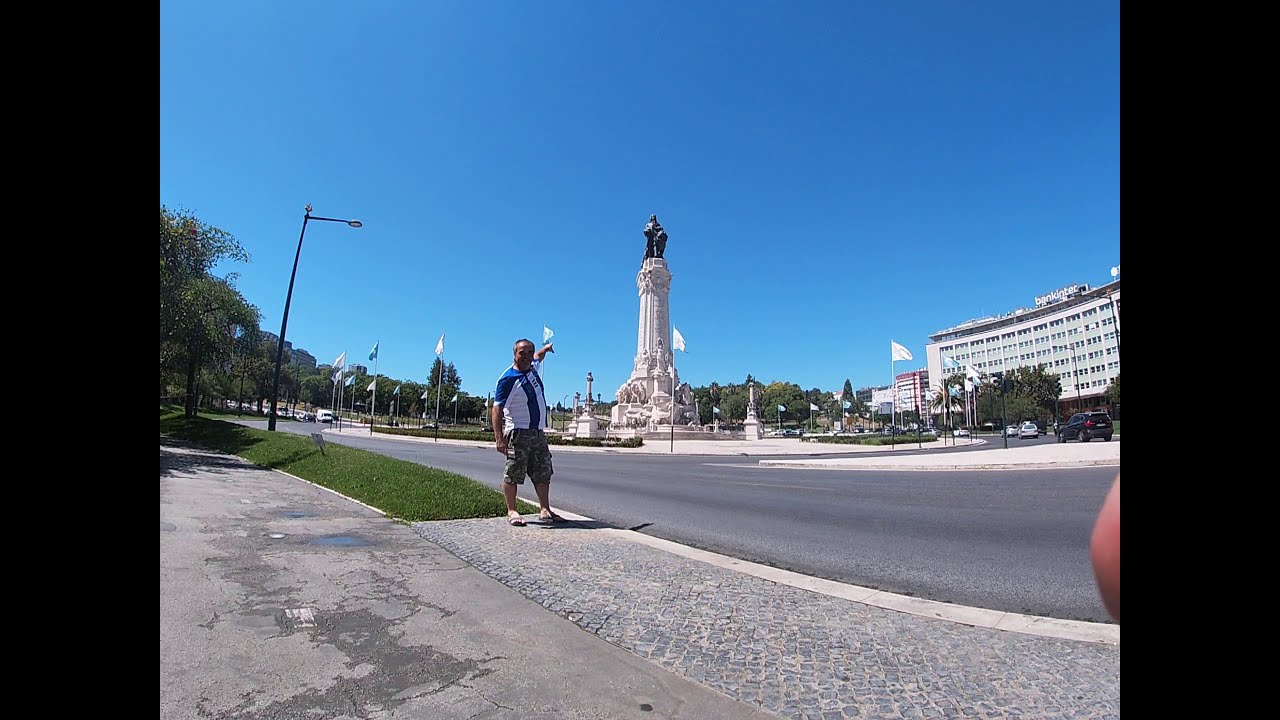The image features a bustling town area with a prominent seven-story building labeled "Bank & Tech" at its center. Situated prominently in the image is a large, intricate monument adorned with multiple black statues, crowned by a significant figure at its peak. Surrounding the monument, multiple cars navigate a roundabout, adding to the city's dynamic atmosphere. The scene depicts a clear, daytime sky with a few scattered clouds, enhancing the vibrant colors of the environment: gray pavements, green trees, blue and white hues, and various shades from tan to red.

Running alongside the road is a crisp walkway flanked by patches of grass, with a man standing on the sidewalk. This man, wearing a white and blue striped shirt, cargo shorts, and sandals, points towards the monumental statue, drawing attention to its grandeur. Across the street, the "Bank & Tech" building, with its many windows, anchors the backdrop. The scene is enriched by distant trees lining the road and multiple flagpoles adding an element of civic pride. Puddles and cracks are visible in a nearby parking lot, indicating recent weather or wear. Overall, the image captures the intersection of urban life, historical grandeur, and natural elements seamlessly intertwined in a vibrant town setting.